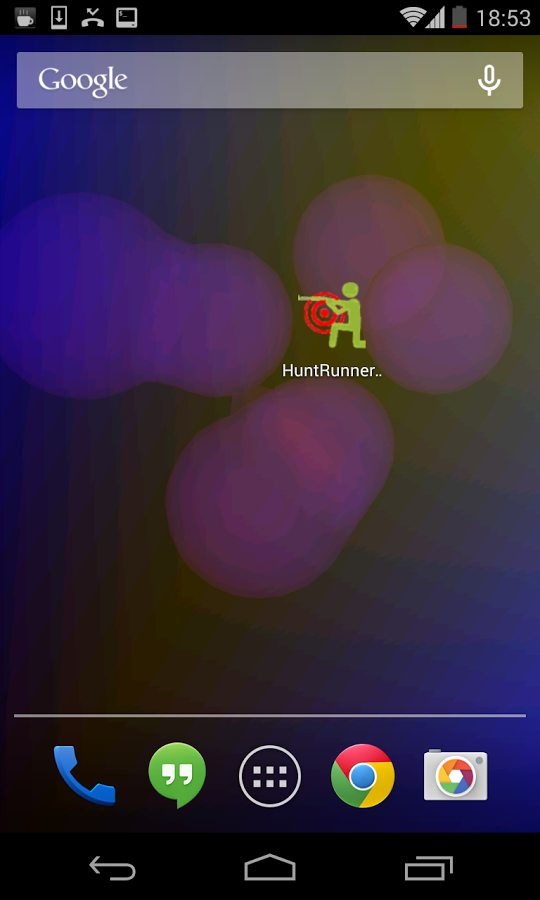The image showcases a mobile device's home screen. At the bottom of the screen, there is a navigation bar containing a back arrow, a home button, and a multi-tab button. The status bar at the top-left corner displays several icons: a coffee cup, a download symbol, a phone signal indicator, and in the top-right corner, a Wi-Fi symbol and a nearly depleted battery icon in red. The time is displayed as 18:53.

The wallpaper background is simple, with the word "Google" in white and a microphone icon to its right. There is a single app icon labeled "Hunt Runner" on the screen. Below that, a row of frequently used app icons is visible, including a telephone, a messaging app, a six-block advanced options icon, the Google Chrome logo, and a camera icon with Google colors integrated into the camera's design.